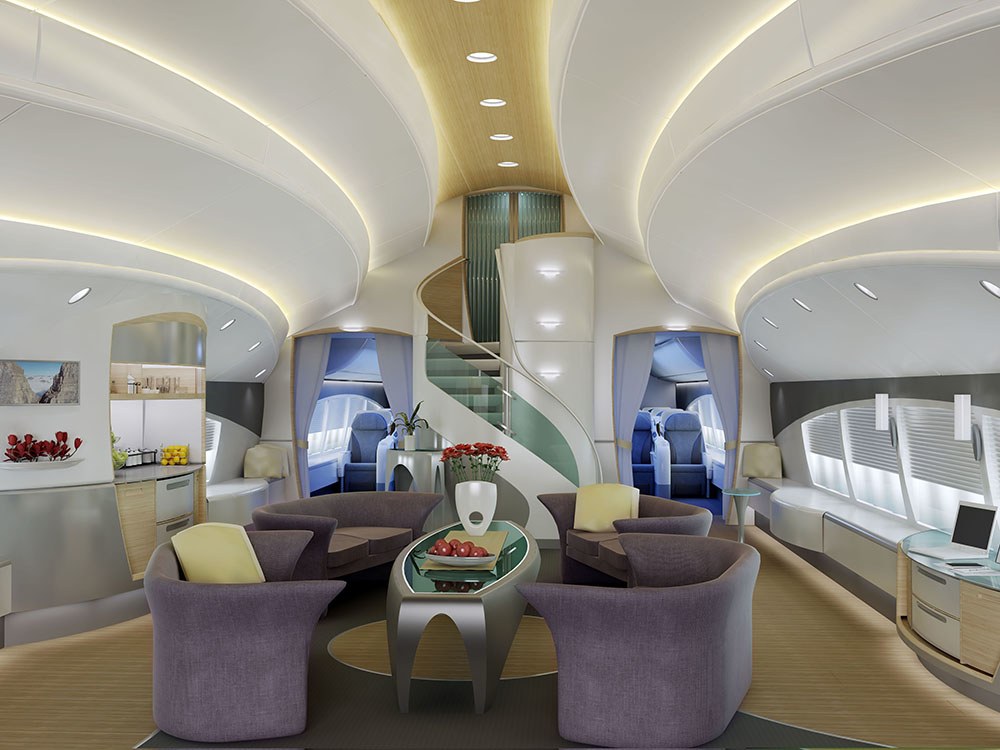The photograph features an opulent first-class section of an airplane, designed with a modern aesthetic that exudes luxury. Central to the image are four modernist purple two-seat sofas, arranged around a sleek metallic table with a glass top, adorned with fresh fruit and a vase of red roses. The first-class lobby is spacious and brightly lit, amplifying the clarity and elegance of its design. A swirly staircase ascends to an upper level, elegantly positioned in the center. The surrounding decor blends white and neutral tones with hints of light purple, creating a harmonious and stylish environment. Windows on either side allow natural light to flood the space, enhancing its welcoming atmosphere. On the left side, a counter showcases a display of lemons and other miscellaneous items, adding to the refined yet homely ambiance of the setting.